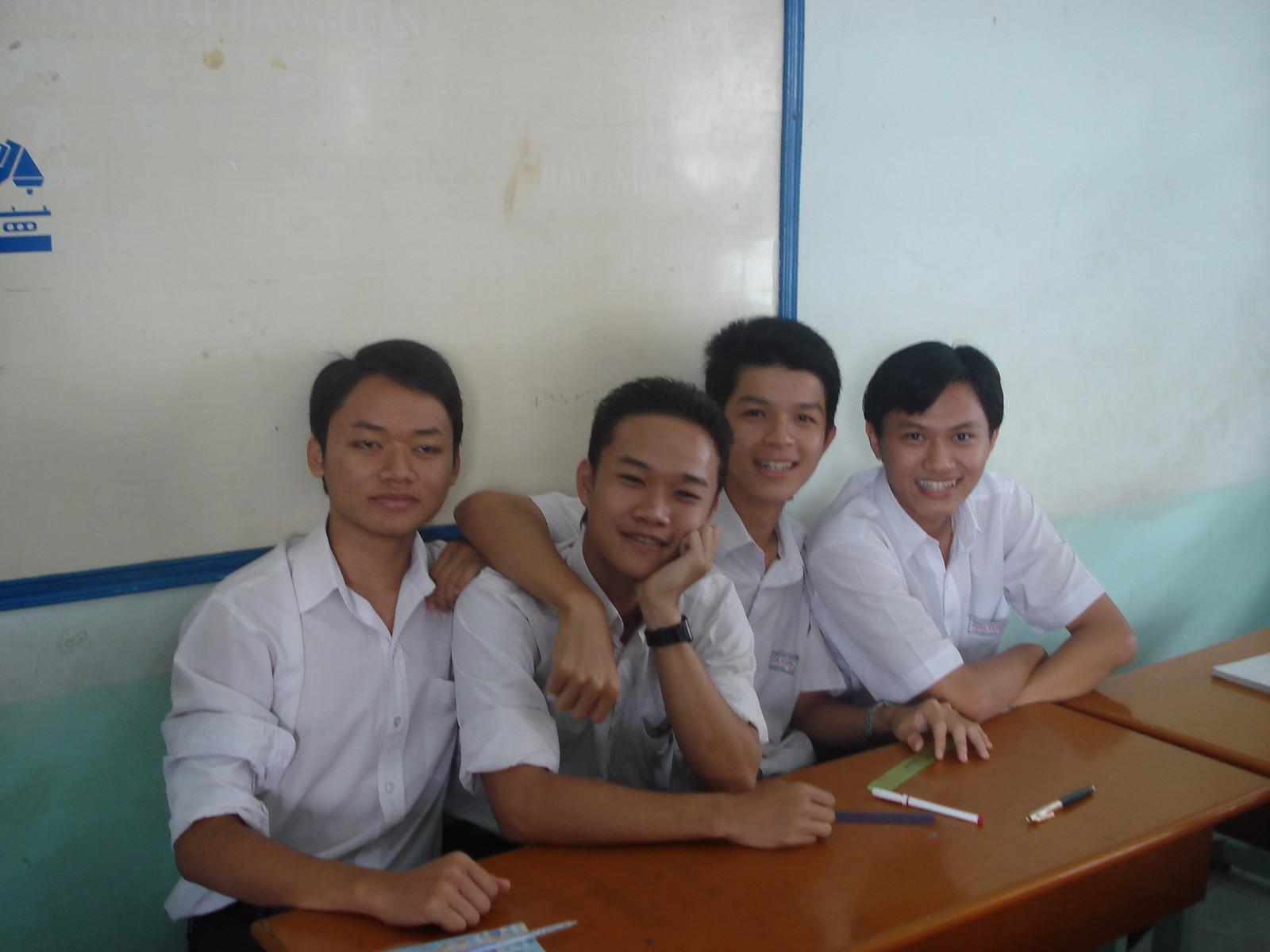This photograph captures four young, possibly Asian men, who appear to be high school or college-age, sitting closely together at a pair of joined wooden desks, in what looks like a classroom. They're all dressed in white button-down shirts with open collars and sleeves that reach just above their elbows, resembling school uniforms. Their camaraderie is evident as a few of them have their arms around each other's shoulders, and they're all smiling, exuding happiness and a sense of friendship. The table in front of them holds various items suggestive of schoolwork, such as pens and a green ruler. The background reveals a whiteboard with a blue border, showing signs of previous use, and a light baby blue wall extending off to the right. Overall, the image conveys a moment of shared contentment and camaraderie, possibly during a break from studying or an in-class activity.